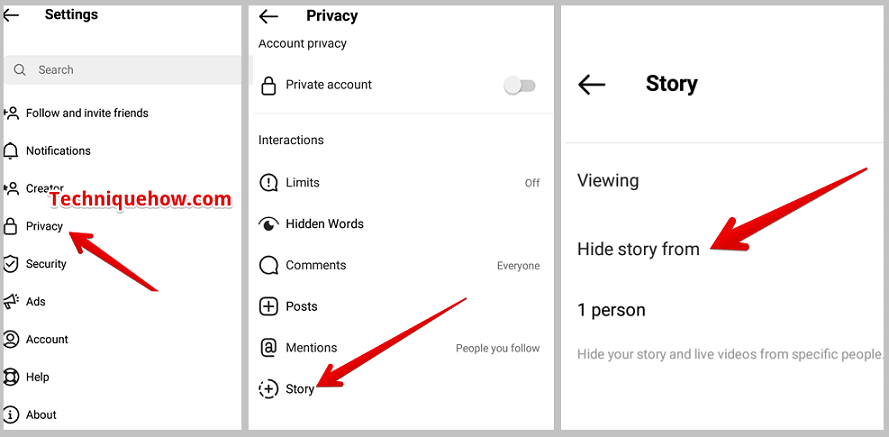The image is divided into three sections. 

**Section 1: Settings Overview**
- This section contains a comprehensive list of settings options, each represented by a unique icon. At the top is a search bar.
  - **Follow and Invite Friends**: Illustrated with an image of a person.
  - **Notifications**: Represented by a bell icon.
  - **Creator**: Similar to the first icon, depicting an image of a person.
  - **Privacy**: Symbolized by a lock.
  - **Security**: Shown as a badge with a check mark.
  - **Ads**: Icon resembling a megaphone.
  - **Account**: Displayed as a circle with a person.
  - **Help**: Depicted with a box inside a circle.
  - **About**: Represented by an eye inside a circle.
- The phrase "techniquehow.com" is prominently written in red within this section, along with a red arrow pointing towards the privacy icon.

**Section 2: Privacy Settings**
- This section focuses on account privacy settings and interactions.
  - **Account Privacy**: Controlled via a slider switch, currently in the "Off" position, accompanied by a lock icon.
  - **Interactions includes the following options**:
    - **Limits**: Option is turned off.
    - **Hidden Words**: No option provided.
    - **Comments**: Set to "Everyone".
    - **Posts**: No option provided.
    - **Mentions**: Two options stated:
      - **People You Follow**
      - **Story** set to "Everyone" with a red arrow pointing from "Everyone" to "Story".
    - Another red arrow directs attention towards the privacy section here as well.

**Section 3: Story Settings**
- This section handles story visibility settings.
  - **Hide Story From**: Linked to a specific person through a red arrow.
  - Describes how to hide stories and live videos from particular individuals.

Overall, the image provides a detailed visual and textual representation of an application’s settings related to privacy, notifications, account management, and story visibility, highlighting specific elements and their respective icons.